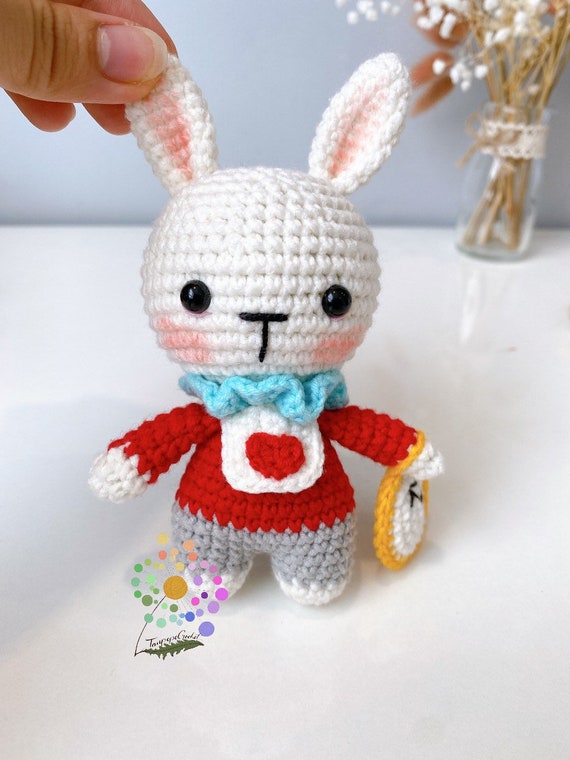This image features a small, crocheted bunny rabbit that is predominantly white with touches of pink blush on its cheeks and inside its tall ears. The bunny has glossy black eyes and a T-shaped black nose and mouth. It is adorned in a blue, fluffy collar around its neck, a red long-sleeved shirt, a white apron with a red heart on the front, and gray pants. A white and gold-rimmed clock is attached to its wrist. The bunny is positioned on a shiny white table surface within a rectangular indoor photograph. In the upper left corner, a woman's thumb and fingers are gently holding the bunny's left ear to keep it upright. Behind the bunny, to the right, there is a glass vase containing brown sticks topped with small, white cotton tufts. Additionally, there is a colorful, circular flower drawing on the bottom left side of the table that spans various colors from green to blue and is signed at the bottom, although the signature is not legible. The background consists of a light blue-painted wall.